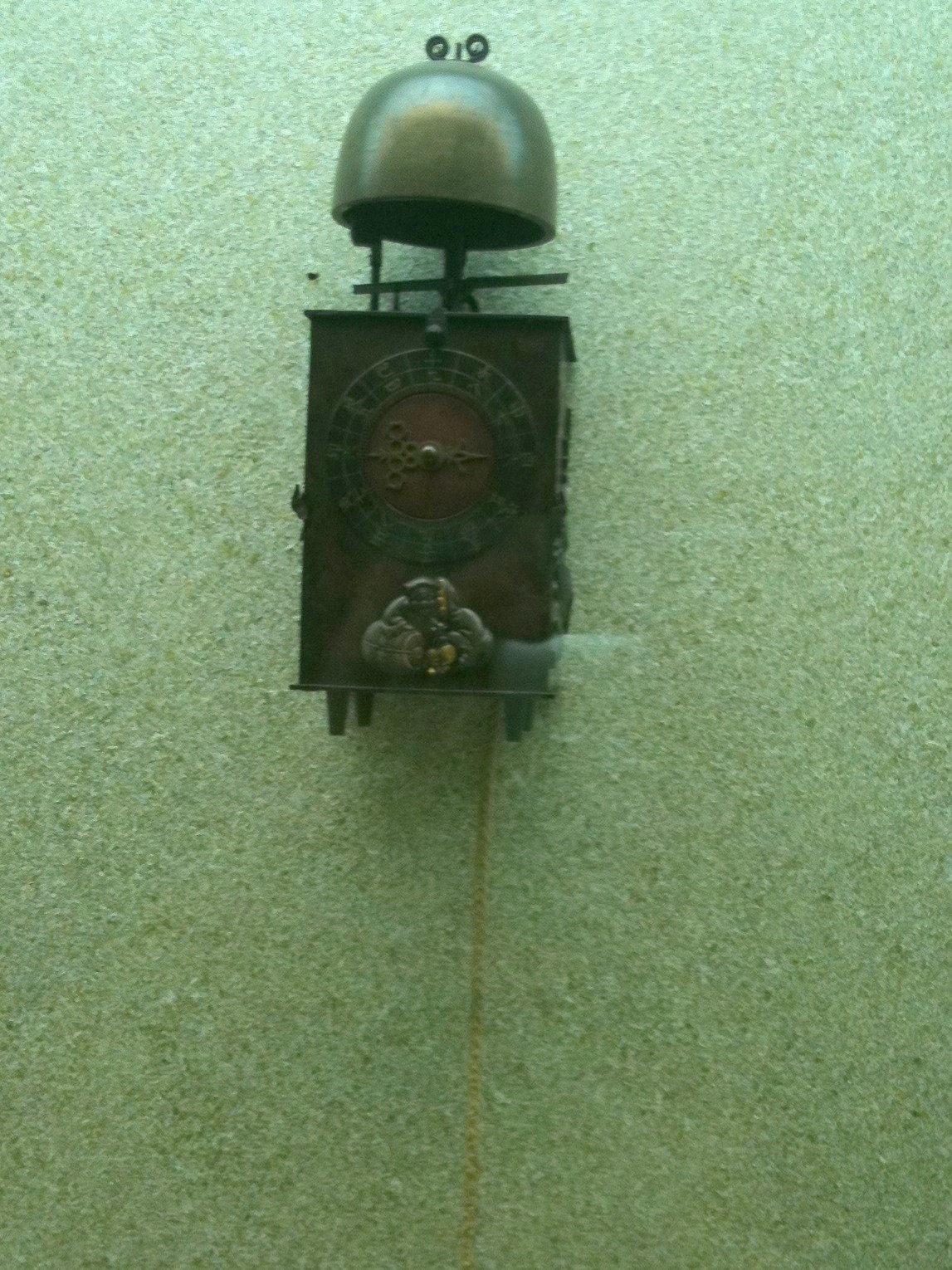The image features a very old-fashioned, antique alarm clock mounted on a wall. The clock itself is a dark mahogany rectangular box with a black circular face in the center, accented with thin, gold-colored hands. Surrounding the clock face is gold lettering on the dial. Above the clock, there’s a large, grayish, dome-shaped bell with two ornate swirls protruding from its top and a cross beam beneath it. The clock stands on four pin-shaped feet and has a faint yellow-gold cord descending from its bottom. The backdrop is a consistently light-gray, rough-textured wall. An orange line runs vertically up the wall, reaching the base of the clock, possibly indicating its alignment or purpose. The overall impression is of a meticulously crafted antique piece, possibly used as an old alarm or thermometer, attached to machinery or a boiler from a bygone era.